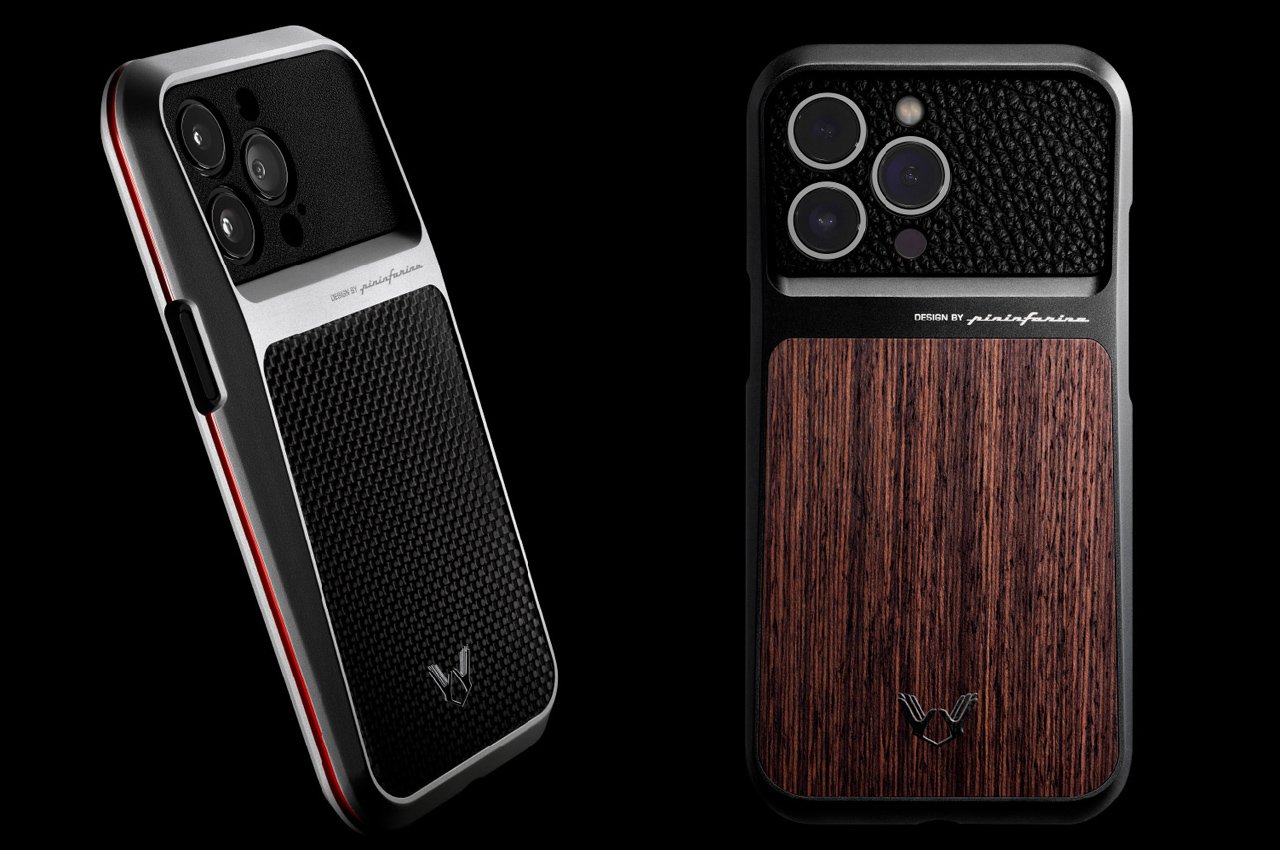The image features two distinct iPhone cases set against a solid black background, each prominently showcasing design elements and brand insignia. On the left is a case with a sleek combination of silver and black, resembling an old speaker or microphone, reinforced with a dark gray mesh pattern and an elegant insignia at the bottom center. The case accommodates the standard trio of camera lenses and a flashlight area. On the right is another iPhone case variant that combines silver and black but stands out with its refined wood grain paneling beneath the camera section. Both cases bear the inscription "Designed by Pininfarina," though the text is slightly difficult to read. The logo on each case, shaped like wings or a stylized 'W,' adds a touch of sophisticated branding to the overall design.